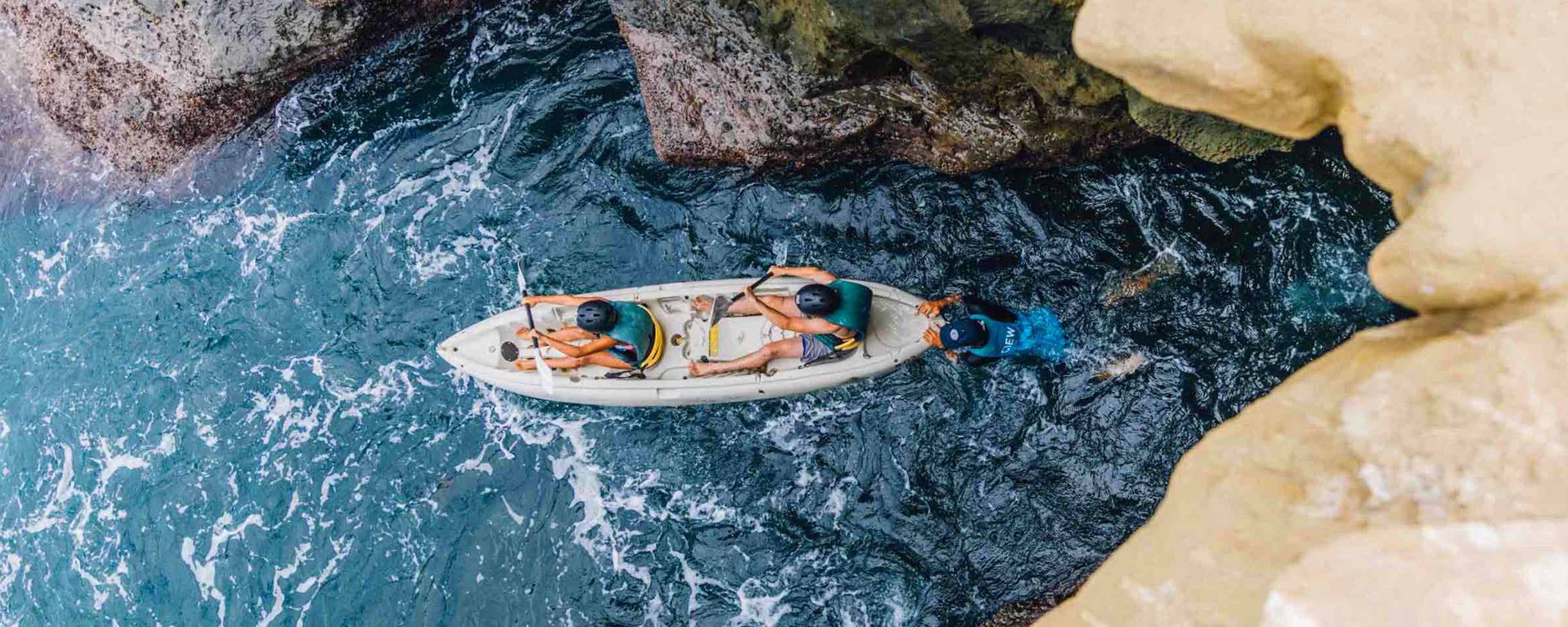The image depicts a bird's eye view of a rugged, rocky crevasse with contrasting light and dark rock formations. At the center, there is a white canoe or kayak carrying two people. The individuals, a man and a woman, are both wearing blue life jackets and shorts, paddling through what appears to be rough water. The man and woman are seated in the boat while holding paddles, seemingly rowing to the right side of the image. 

In addition, a third person is visible in the water behind the boat, pushing it with both hands. This individual is also equipped with a blue life jacket and a helmet. The water has a dark hue on the right side, transitioning into a lighter layer on the left. The rocks framing the scene are dark gray-black towards the top edge and appear smoother and worn near the bottom and closer to the viewer, giving a sense of depth and perspective. The photo is horizontal and rectangular, emphasizing the dramatic, overhead view of the scene.